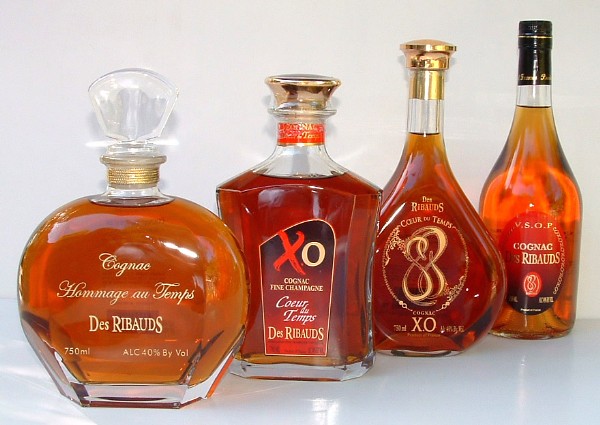The image features four distinctive bottles of cognac meticulously arranged in a diagonal formation on a white table, accentuating their differences against the stark background. Each bottle, sealed and untapped, showcases a variety of cognac from the brand De Ribot, bearing the label "Cognac Hommage au Temps." The arrangement progresses from the shortest bottle at the front to the tallest at the back, creating a dynamic visual.

Starting from the left, the first bottle is rounded with an ornate, crystal stopper, containing a light brown liquid. Its label mentions the brand De Ribot and the specific variety "Hommage au Temps," along with details like 750 milliliters and 40% alcohol by volume. Next, a rectangular, tapered bottle also features a glass top and gold writing, marked with "X O," indicating a fine champagne cognac. The third in line is a rounded bottle that tapers upward, with a gold cap and similar decorative elements, labeled "Cour du Temps" and "XO." Finally, the bottle at the far right is more traditionally shaped, adorned with the designation "VSOP" and topped with a black cap.

Each bottle contains the characteristic light brown hue of cognac, providing a cohesive yet varied display of this distinguished spirit.